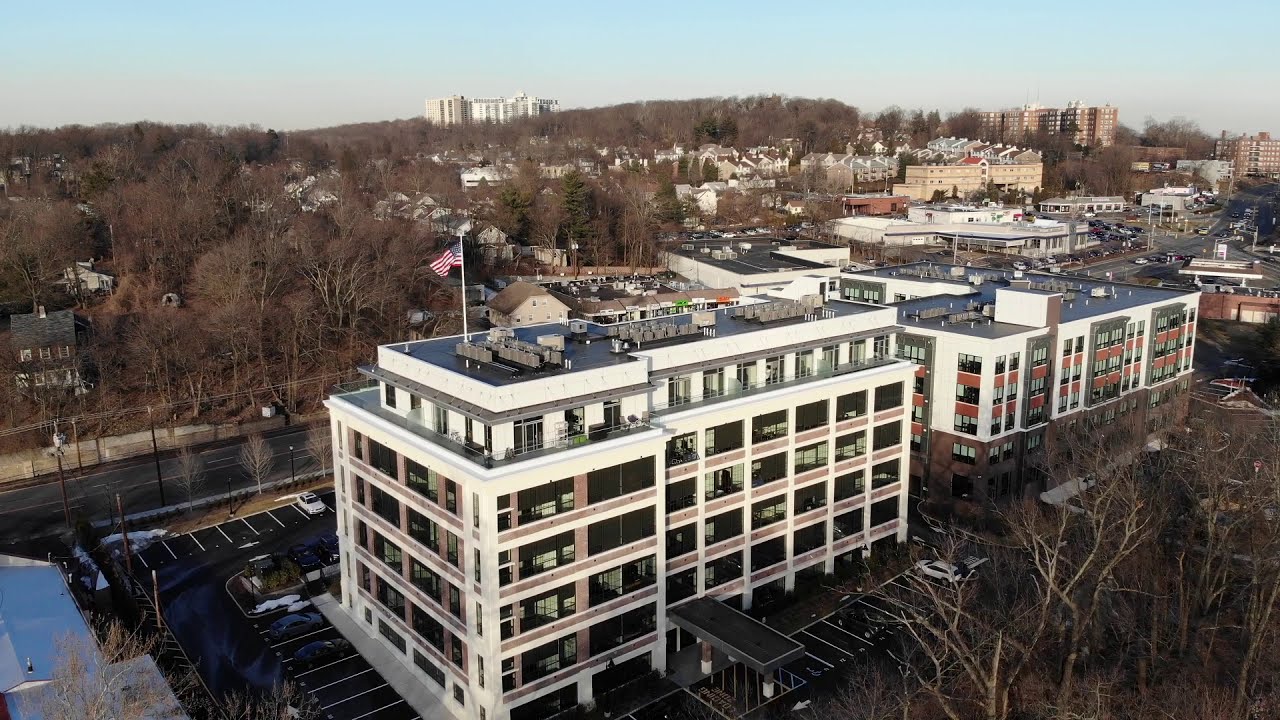This detailed image depicts an overhead view of a suburban cityscape centered around two prominent apartment buildings. The left building stands out with its white exterior, gray and black rooftops, and a striking reddish siding, topped with an American flag on a white pole. Its neighboring building is slightly shorter, four stories tall, also painted white but featuring orange accents. Both are enveloped by a sprawling blacktop parking lot with clearly marked white parking spaces. Vehicles of various colors, including white, black, and gray, are scattered throughout the lot.

Surrounding these buildings, a network of streets with traditional blacktop and marked white or yellow lines runs through the area. The season appears to be winter, as indicated by the bare brownish-gray trees devoid of leaves. In the middle ground, a lone white house with a gray rooftop peeks out from behind the left apartment. Further in the back, the skyline is dotted with buildings of various hues—white, tan, orange, and brown—providing a rich tapestry of architectural styles against a blue sky.

The picture, likely taken from an elevated point such as a drone or a taller building, showcases not just the immediate structures but also the sprawling urban environment continuing into the distance, highlighted by additional apartment buildings, houses, and a busy main street with moving traffic. In the extreme background sits a prominent tall building, perched on a hill, completing the diverse and expansive view of this suburban city.